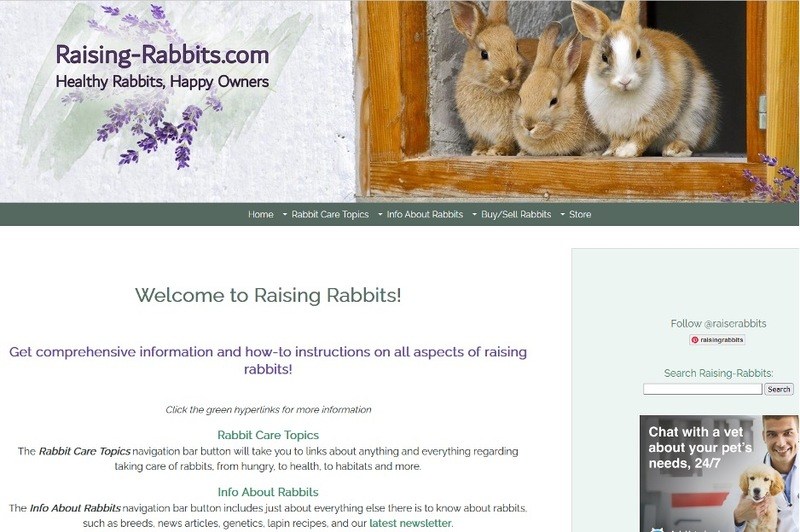**Screenshot Description: Website Overview for Raising Rabbits**

The screenshot showcases the homepage of the website "RaisingRabbits.com." Prominently featured are three adorable bunny rabbits, mainly brown with some white markings. One rabbit in the center has a striking half-and-half brown and white coat. 

The website's logo and header banners a welcoming message: "Healthy Rabbits, Happy Owners." The navigation bar sits below, featuring the tabs: Home, Rabbit Care Topics, Info About Rabbits, Buy/Sell Rabbits, and Store.

The main content highlights a comprehensive resource for rabbit care, offering detailed insights on all aspects of raising rabbits. Visitors are encouraged to explore further by clicking green hyperlinks. In the highlighted "Rabbit Care Topics" section, mentioned in a green font, the navigation bar button is designed in black. This section leads to links covering a wide array of rabbit care topics, including feeding, health, habitats, and more.

Similarly, the "Info About Rabbits" section, also featured in green text, is accessible through a black navigation bar button. This section provides extensive information about rabbit breeds, news articles, genetics, and recipes for rabbit meat ("LAPIN").

This detailed and user-friendly layout ensures that rabbit enthusiasts can easily navigate through the wealth of information available on the site, making it a valuable resource for both novice and experienced rabbit owners.